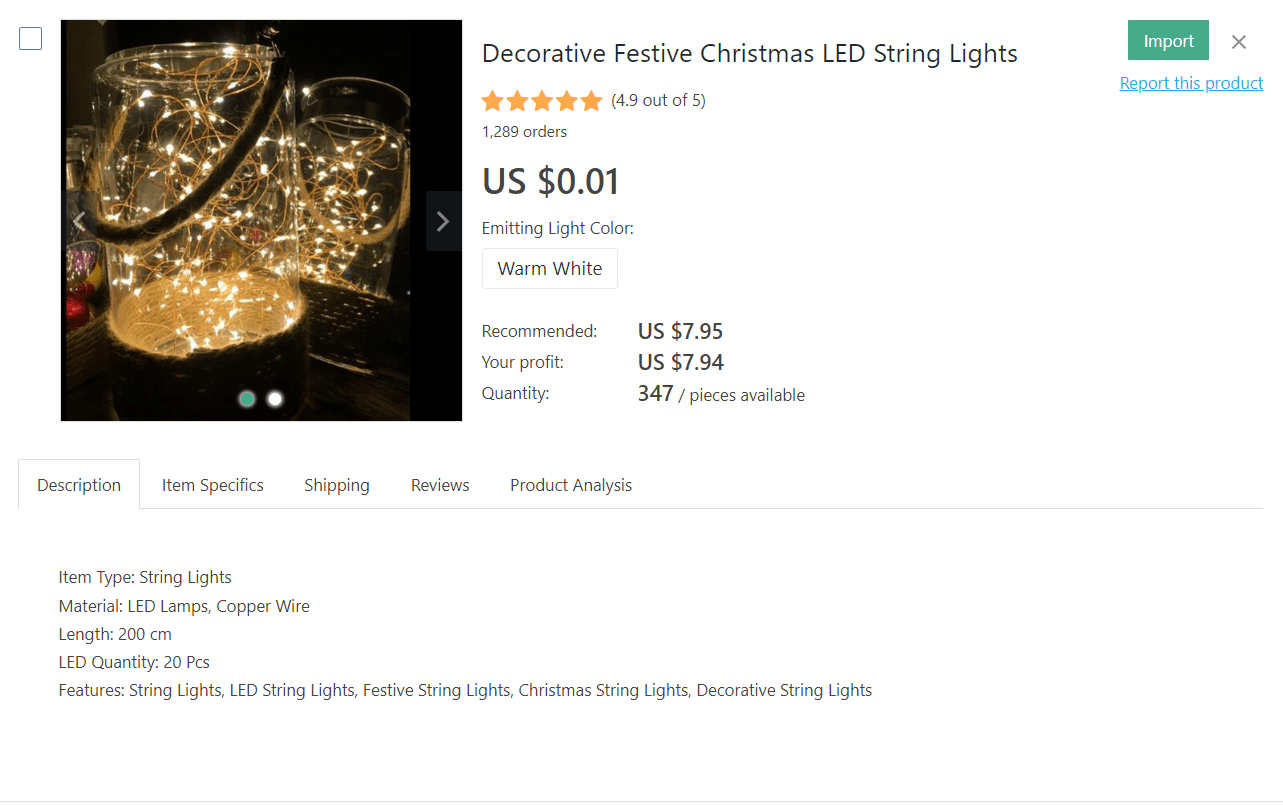**Detailed Caption:**

The image displays a promotional screenshot from a website offering Decorative Festive Christmas LED String Lights. A clear glass jar is showcased, illuminated by a coiled string of fine, warm white LED lights, creating a cozy and enchanting atmosphere. These string lights are typically powered by a series of AA or AAA batteries connected to a small battery case, making them versatile and perfect for festive decor.

The promotional details on the website highlight an exceptional offer, where the US price is listed as $0.01 per unit with a recommended retail price of $7.95, promising a significant profit margin of $7.94. The inventory boasts an available quantity of 347 pieces.

The comprehensive description provided includes item specifics and features such as:
- **Item Type:** String Lights
- **Material:** LED Lamps, Copper Wire
- **Length:** 200 centimeters
- **LED Quantity:** 20 pieces

This product is ideal for creating festive, decorative accents in jars, around the home, or at events, with key features emphasizing its use as string lights, LED string lights, festive string lights, Christmas string lights, and general decorative string lights.

The screenshot also details various aspects like shipping, reviews, and product analysis, giving potential buyers all the information they need to make an informed purchase.